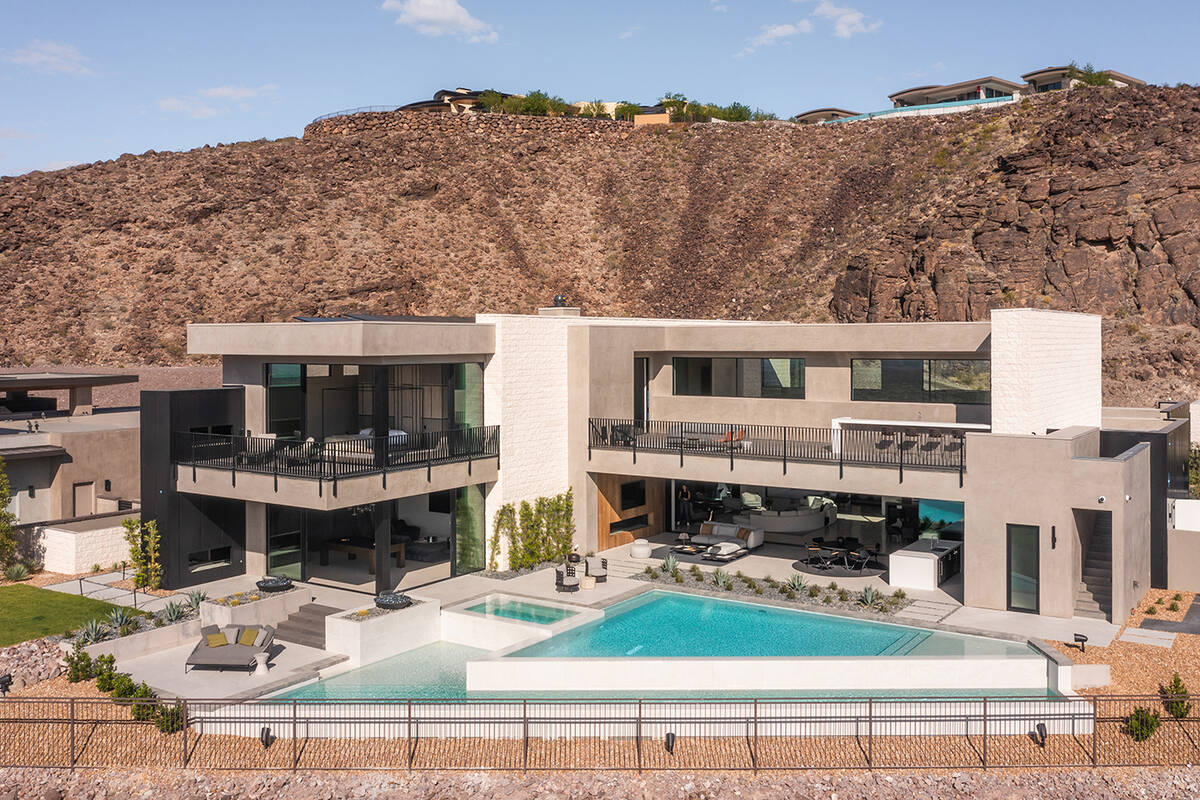The image captures a modern, two-story house set in a desert valley under clear blue skies with a few scattered clouds. The backdrop consists of a brown, rocky hill with a few houses perched on top. The house itself is large and extends horizontally across the picture, with a beige and white exterior that emphasizes its minimalist, angular design, characterized by its flat roof and extensive use of glass and concrete.

In front of the house is a spacious area with a considerable pool and a separate jacuzzi on the left side. The right side of the image reveals open outdoor spaces that resemble an open living room and an open bedroom, emphasizing the house's open-concept, modern architecture. There is also a metal gate stretching from left to right in front of the property, while a roof deck can be seen on the right side of the house. The environment is predominantly rocky with sparse vegetation, mainly small bushes, contributing to the overall minimalistic and somewhat stark aesthetic of the scene.